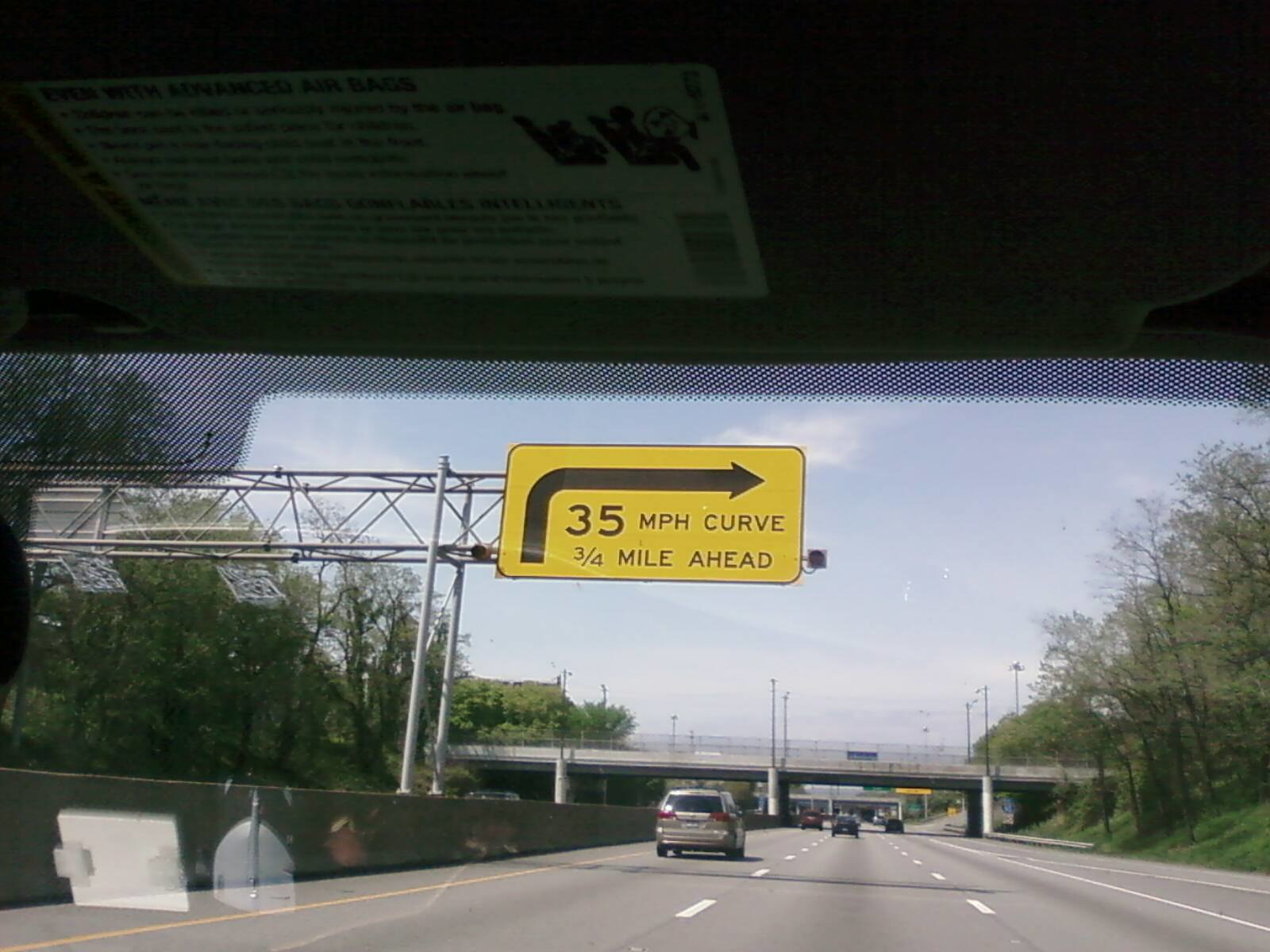A photograph taken from inside a vehicle captures a scene through the windshield. The upper portion of the image prominently shows a sun visor equipped with a white sticker featuring indistinguishable black writing due to shadows. The lower part of the photograph reveals the view through the windshield, slightly obstructed by reflections of plastic items on the lower left corner. The setting is a four-lane highway, with the vehicle traveling forward in the right lane. In the left lane, a gray SUV can be seen. Ahead in the distance, an overpass looms over the road. The focal point of the image is a bright yellow street sign indicating a 35 mile per hour curve three-fourths of a mile ahead, with a black arrow pointing to the right.